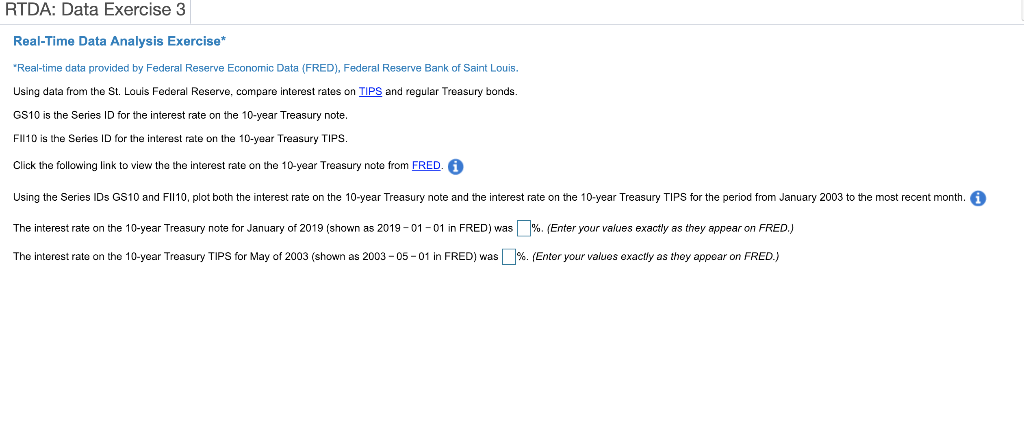The image displays a printed document titled "RTDA Data Exercise 3" at the top left in black text. Below this, in blue print, it reads "Real-Time Data Analysis Exercise*" with an asterisk indicating that the data is provided by the Federal Reserve Economic Data (FRED) from the Federal Reserve Bank of St. Louis. 

The text on the document outlines an exercise that involves using data from the St. Louis Federal Reserve to compare interest rates on Treasury Inflation-Protected Securities (TIPS) and regular Treasury bonds. The term "TIPS" is highlighted in blue, making it a clickable link. 

Further instructions specify that the series ID for the interest rate on the 10-year Treasury note is "GS10," while the series ID for the interest rate on the 10-year Treasury TIPS is "FII1." The document instructs users to click a provided link to view the interest rate on the 10-year Treasury note from FRED and to use the series IDs "GS10" and "FII10" to plot both interest rates from January 2003 to the most recent month.

The document includes fields where users should enter the interest rate data as it appears on FRED. Specifically, it instructs users to fill in the interest rate for the 10-year Treasury note for January 2019 (shown as "2019-01-01" in FRED) in an empty box for percentage. It also asks for the interest rate for the 10-year Treasury TIPS for May 2003 (shown as "2003-05-01" in FRED) in another empty box for percentage. Users are reminded to enter their values exactly as they appear on FRED.